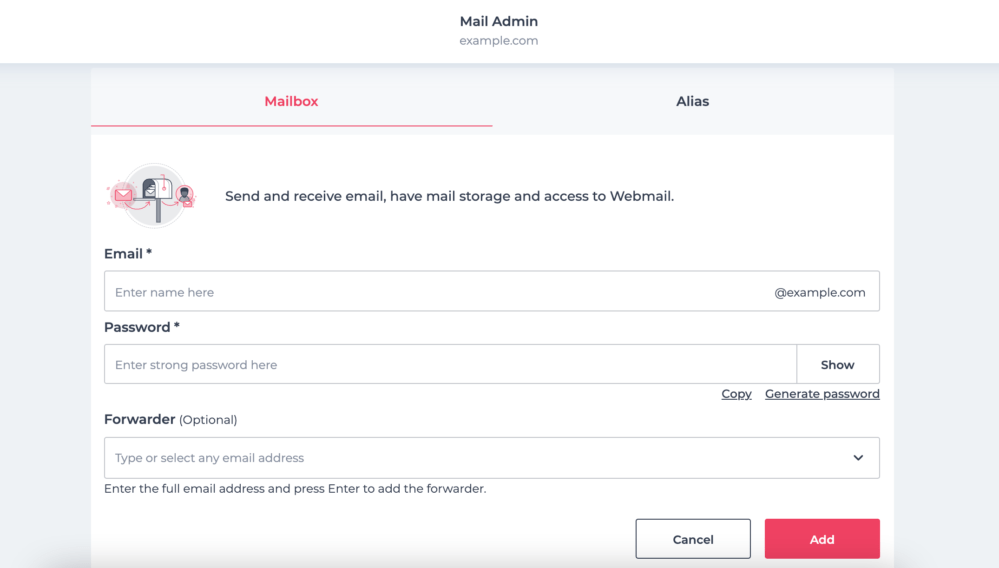The image centers around a screenshot of an email administration interface. At the very top, the bold text "Mail Admin" is displayed, followed by the domain "example.com" in a fainter gray. Directly beneath, the interface transitions into a light gray background where a white rectangular tab showcases two top navigation options. The first tab, labeled "Mailbox" on the left, is highlighted in red, indicating the current active selection, while the second tab, "Alias," appears in gray.

Directly below this, on the left, is an icon depicting a mailbox with a red envelope being inserted and pulled out, alongside an arrow pointing towards a person icon accompanied by a small envelope at its base. Adjacent to this graphic is a description text that reads: "Send and receive email, have mail storage, and access to webmail."

Proceeding further down, the interface starts presenting input fields and options. The first input field is labeled "Email" with a mandatory asterisk, suggesting users enter an email prefix next to the preset domain "@example.com." The next field prompts users to input a "Password," also marked with an asterisk to denote its required nature. To the right of this, there is a divided button featuring the word "Show," which likely functions to reveal the obscured password for verification purposes.

Below the password input, the interface offers two highlighted buttons: one displaying the option to "Copy" the password, and the other to "Generate Password." Moving further down, there is an additional optional field labeled "Forwarder." This drop-down menu allows users to "Type or select any email address." Directly below, instructions advise users to "Enter the full email address and press enter to add to the forwarder."

Finally, situated in the bottom right corner are two rectangular buttons. The gray button, inscribed with "Cancel" in white text, offers an option to exit the process, whereas the red button, stating "Add," solidifies the selected configurations.